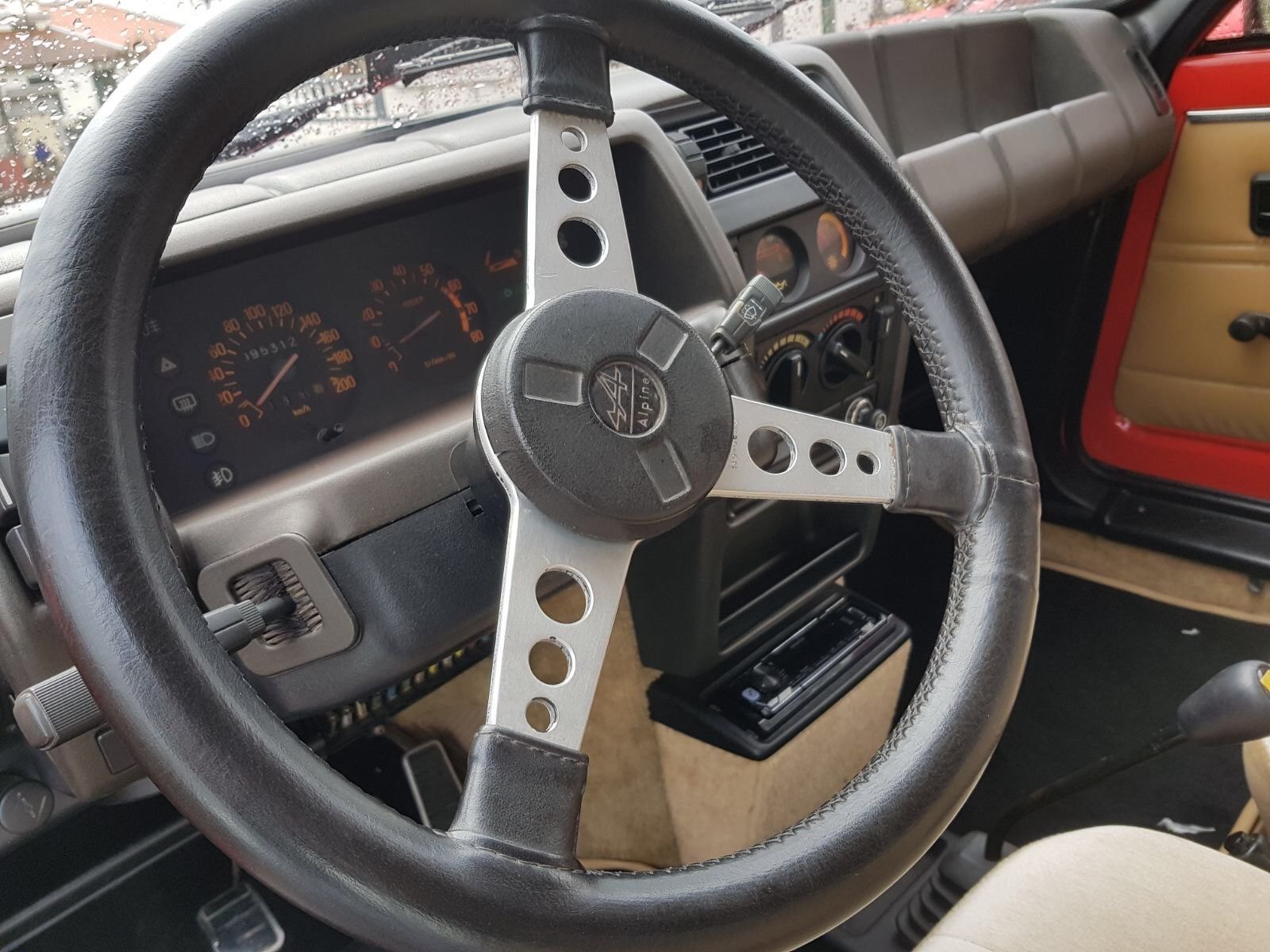The image is a color photograph taken from the driver's seat highlighting the interior of an old car, possibly from the 1980s. The car's dashboard and interior feature a mix of gray and tan leather surfaces, with a touch of brown and red accents on the doors. The dashboard is adorned with analog instruments, including a speedometer and a fuel gauge, emphasizing its vintage look. A radio is positioned unusually low, resembling the placement of an ashtray, and it's facing upwards from the center of the dash. The steering wheel, prominently centered in the image, is wrapped in black leather and features a steel, tri-pronged design. Below the steering wheel, a stick shift protrudes from the floor, indicating the vehicle has a manual transmission. The door visible on the right side showcases tan leather, rimmed with red leather, and includes a manual window mechanism. The windshield displays raindrops, and through it, a building with a red roof is faintly visible. Overall, the car's antiquated features and lack of modern digital elements underscore its vintage charm.